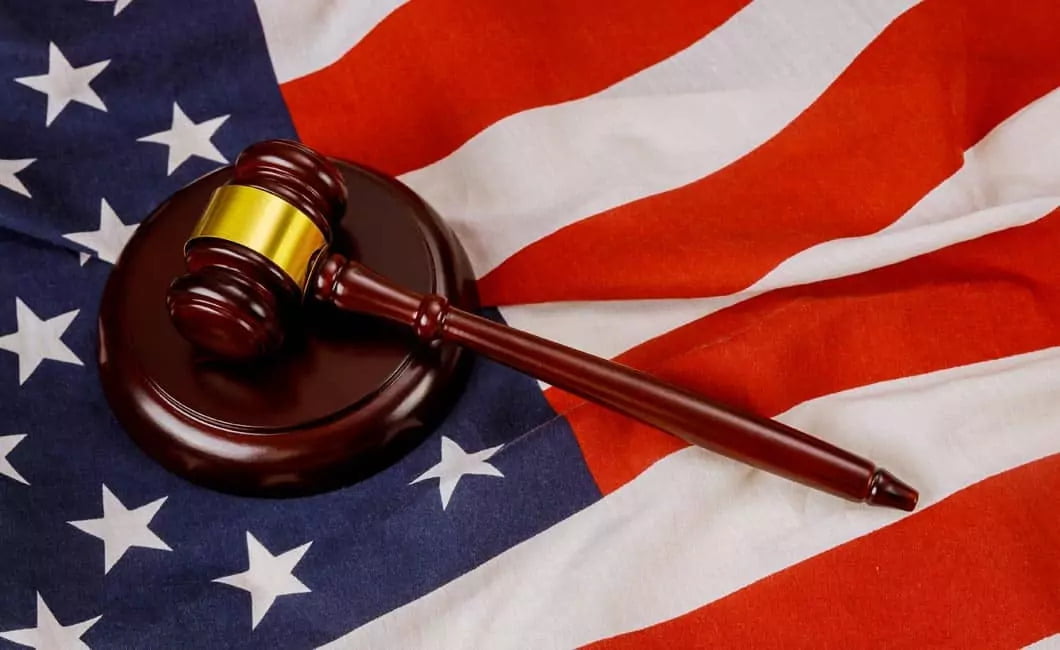This detailed photograph captures a close-up of a partially visible, slightly rumpled American flag lying flat. The flag's blue canton, adorned with white stars, lies to the left, while the red and white stripes stretch towards the right. Dominating the scene is a polished, cherry-wood colored judge's gavel, laid diagonally across the flag. A prominent gold band encircles the middle of the gavel's head, adding a striking contrast. The gavel rests upon a circular sound block, which is positioned on the blue section of the flag, covering some of the stars. The wood of the sound block and gavel appears shiny and reflective, adding an element of depth to the image. This composition juxtaposes symbols of justice and national identity, encapsulated within the rich textures and colors of the materials.